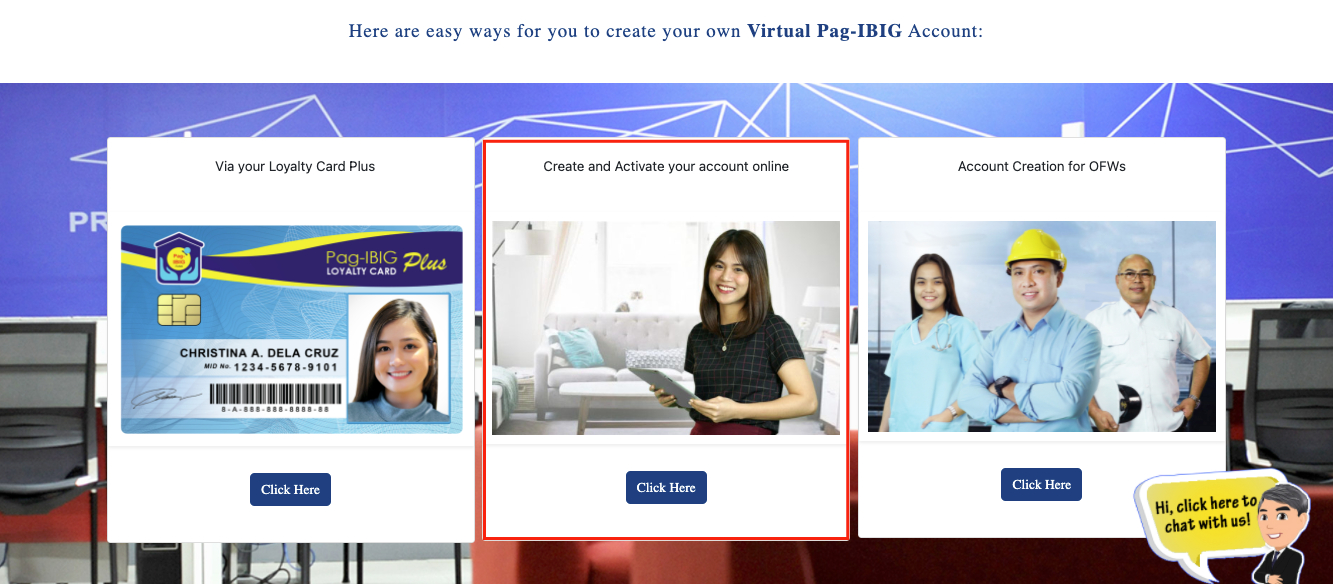This digital image serves as a guide for creating and activating a virtual PAG-IBIG account using the Loyalty Card Plus. At the top, in bold text, it reads: "Here are easy ways for you to create your own virtual PAG-IBIG account via your Loyalty Card Plus."

At the center, there is a picture of a Loyalty Card featuring a chip, with the name "Christina A. de la Cruz" prominently displayed.

To the left, a smiling Asian woman with dark hair is featured.

On the right side, another woman with dark hair is smiling in a cozy living room setting, holding an iPad. Beneath this image, there's a "Click Here" button and the text: "Create and activate your account online."

Further to the right, a trio of individuals stands together. The group includes a woman and two men, with the man in the center wearing a yellow hard hat and crossing his arms. Above them, the text reads: "Account creation for OFWs."

This image illustrates the various ways to set up a virtual PAG-IBIG account, with detailed steps and representations showing diverse users and scenarios.